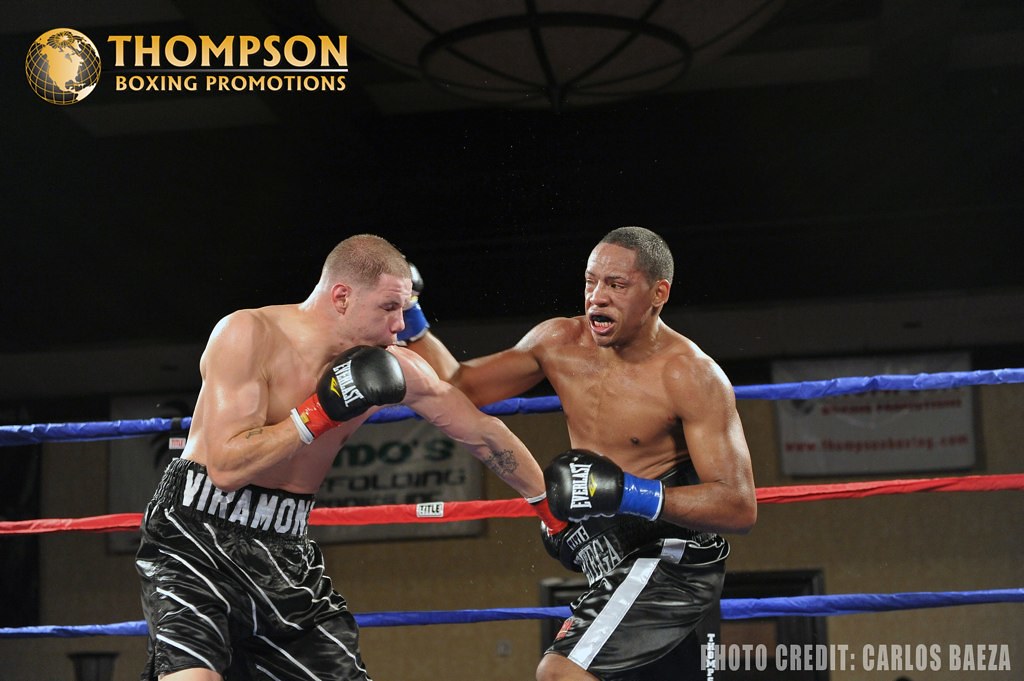The image captures an intense moment in a boxing match between two fighters. The boxer on the left, a white man with short blonde hair, is shirtless and wearing black trunks with silver diagonal stripes and the name "VIRAMON" in gray-silver text. He sports black boxing gloves with red wrist tape and a tattoo on his left forearm. He is seen delivering a downward punch aimed at the waist of his opponent. The boxer on the right, a black man with short black hair, is also shirtless, donning black shorts with a silver stripe. He wears black gloves with blue wrist tape and has a black mouthguard. He is captured in the midst of a punch directed towards the head of the boxer on the left. The boxing ring ropes in the background are configured in blue, red, and blue from top to bottom, tilted slightly downwards from right to left. The background reveals a light brown wall adorned with large plastic signs featuring text in various colors, too distant to discern clearly. High above them, a darkly colored dome descends from the ceiling, contributing to the moody atmosphere of the setting. The logo "Thompson Boxing Promotions" in gold with a globe design is visible in the top left corner, and the image is marked by a semi-transparent watermark at the bottom reading "Photo Credit Carlos Baeza."